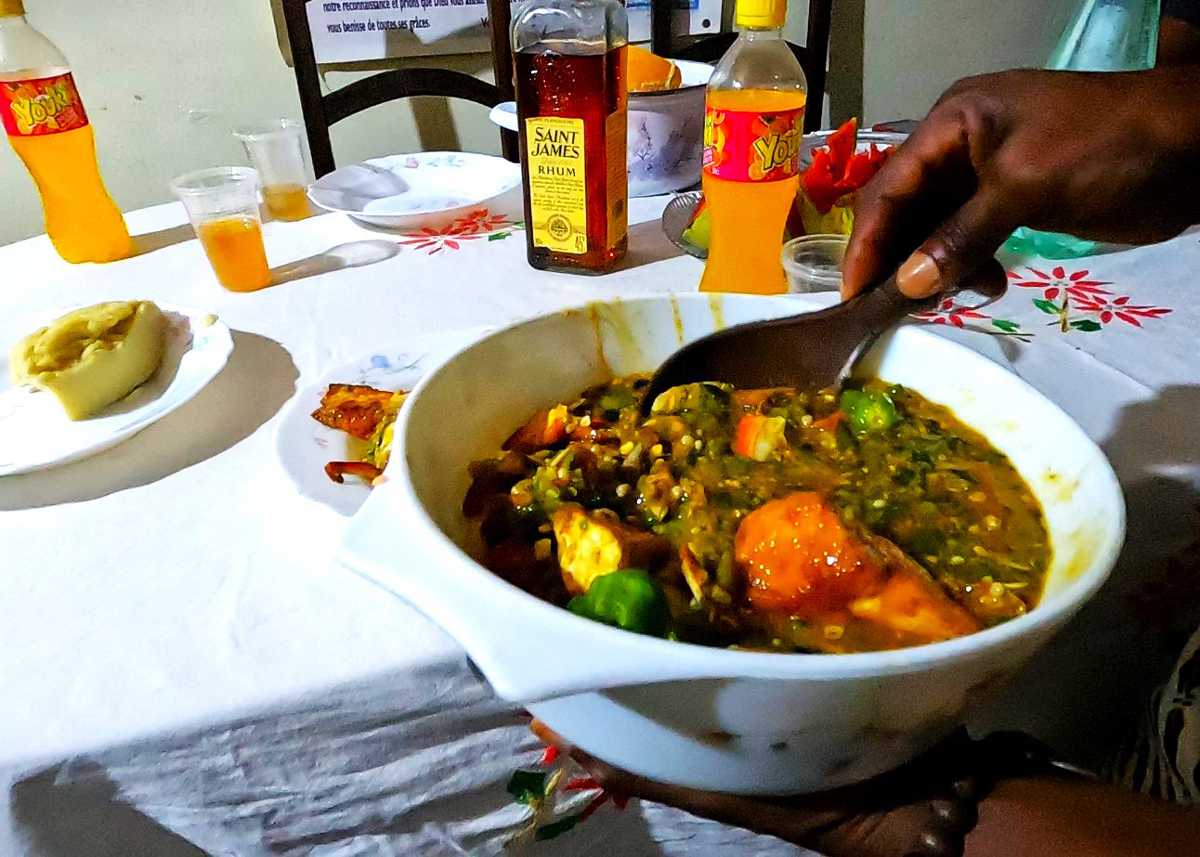This close-up photograph captures an African-American woman holding a large white bowl of what appears to be a vegetable and meat stew with a greenish-red sauce. She is using a brown wooden serving spoon inserted into the bowl, some of the colorful sauce dripping down the sides. The dish contains a variety of vegetables, including okra, and pieces of meat or fish. The table she's standing in front of is covered with a white tablecloth and is set with matching plates, a bottle of St. James rum, two bottles of orange soda, and plastic cups filled with the orange soda. There also appears to be a small pastry or muffin on a smaller white plate, adding to the assortment of items on the table. The scene is vibrant with the multitude of colors from the stew and the well-arranged items, portraying a sense of a communal or festive meal.